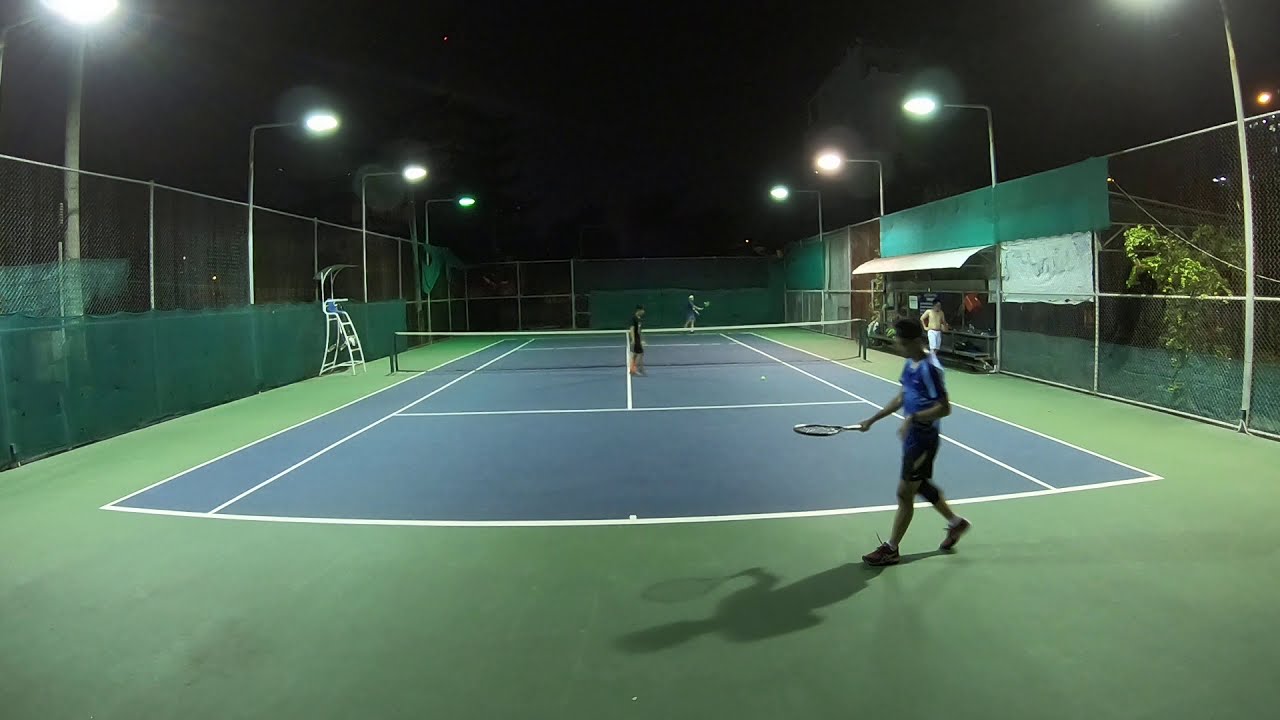The photograph captures a nighttime scene of a tennis court, illuminated by bright overhead lights against a dark sky. The court has a blue playing surface with a surrounding green area and is encircled by a tall chain-link fence. Closest to the camera stands a player in blue, clearly visible, while another player, located at the far end of the court, is too distant to discern any details. A third person is crossing the court near the net, and a fourth individual is positioned on the left side near some bleachers laden with indistinguishable items. The right side of the court, near the net, features shelves and an awning, with a few more people milling about in that area. The vibrant colors and the clear lighting create a vivid depiction of this active nighttime tennis match.